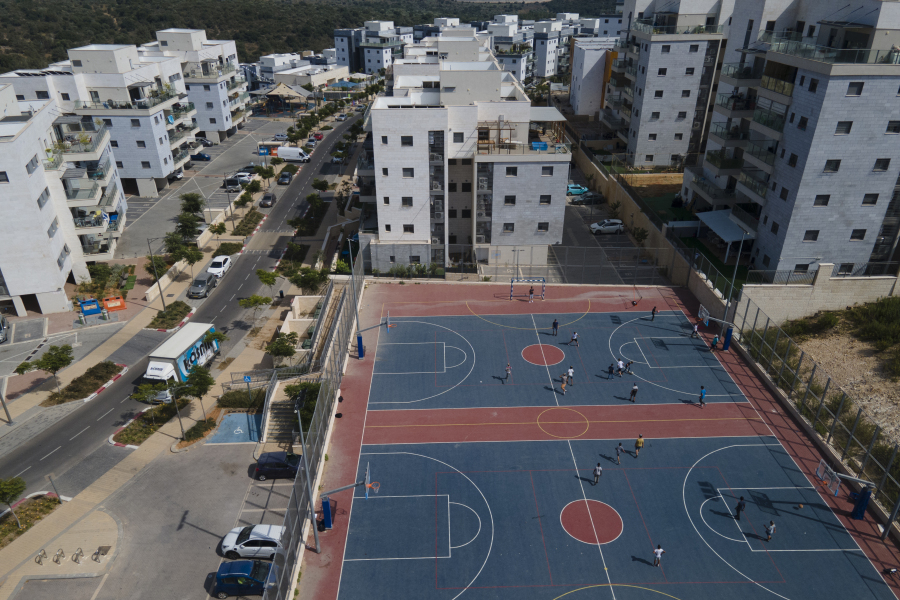This aerial photograph captures a vibrant neighborhood dominated by modern, white-painted apartment buildings that are five to six stories tall. The buildings are rectangular with small, square windows, and some feature balconies with clear glass railings. Centrally located in the image are two large, fenced basketball courts with a distinctive grayish-blue and reddish-brown surface. Despite their primary purpose, it appears that the courts are also being used for soccer, with tiny figures visible playing on them. Surrounding the courts are three rows of boxy apartment buildings, arranged methodically along two parallel streets that cut through the scene. To the right of the courts, there is an empty lot, while on the left, a two-lane road passes by, lined with parked cars. In the background, the urban landscape is framed by towering mountains, contrasting sharply with the meticulously organized city layout below.